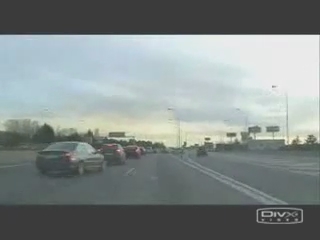This image, a small black-and-white photograph from a vehicle-mounted camera, captures a congested freeway from a low angle. The scene shows a stretch of highway with at least five to seven cars lined up and stopped, indicating heavy traffic. The cars are too washed out to distinguish colors, but a few brake lights are visible. The freeway features dual white or yellow lines and a separate lane of traffic moving in the opposite direction. At the bottom right, a "D-I-V-X" label is partially legible. The overall view is framed by black bands at the top and bottom. Off to the right, an off-ramp extends, and a small building with signs and power lines is visible nearby. In the background, trees and distant streetlights are seen beneath a light, expansive sky filled with white and grey clouds, suggesting an overcast condition or close to sunset.